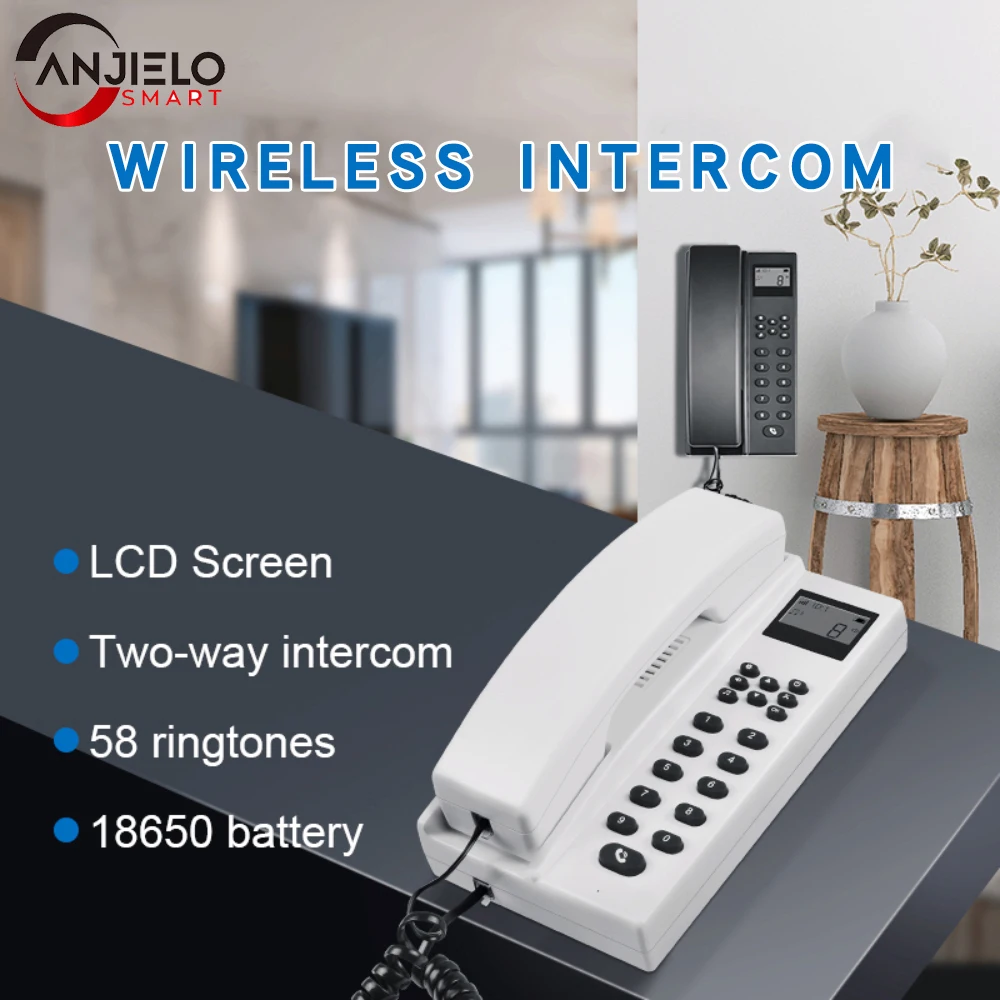This full-color vertically rectangular advertisement features a digitally enhanced, indoor scene with both natural and artificial light. The setting is a blurred room, possibly a kitchen with windows and a chandelier. The focus is on two landline telephones: a white corded push-button phone with a digital display and a black version of the same model mounted on a white wall.

At the upper left corner of the advertisement, the company's logo "Angiello Smart" appears, with "Angiello" in black text, "Smart" in red text, and a partially visible circular design around the letters "ANJ," the top of which is black and the bottom red. Across the top center in large blue text outlined in white, it reads "Wireless Intercom."

At the bottom left, four circular blue bullet points with white text detail the features of the phones: "LCD screen," "Two-way intercom," "58 ringtones," and "18650 battery." The black phone is prominently displayed hanging on the wall above a small wooden table with a vase and plant, while the white phone, appearing to be photoshopped, rests on a grey countertop in the foreground. Both phones have black buttons and cords, further emphasizing the traditional design amidst the modern setting.